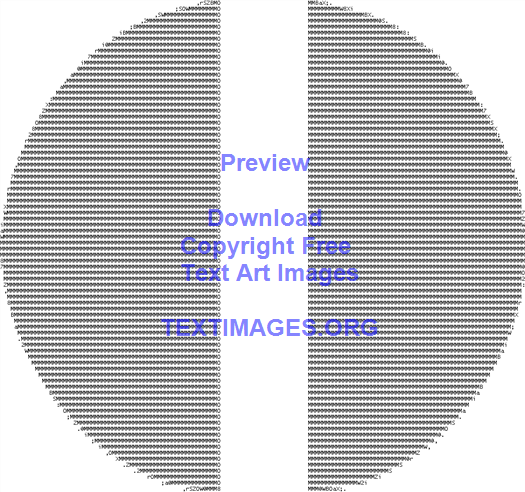The image is a computer-generated printed artwork presenting a striking circular design split into two symmetrical halves. In the middle of the circle, a white line creates a division between the two gray half circles. Each half circle is meticulously crafted from small black geometric pieces, forming an eye-distorting, intricate pattern. Overlaying the center of the artwork, a watermark in light blue text reads: "preview, download, copyright free, text art images, textimages.org." This watermark suggests that the image is a screen capture from a website offering free downloadable images. The overall composition combines geometric artistry with a modern digital aesthetic, emphasizing the availability and accessibility of the artwork.